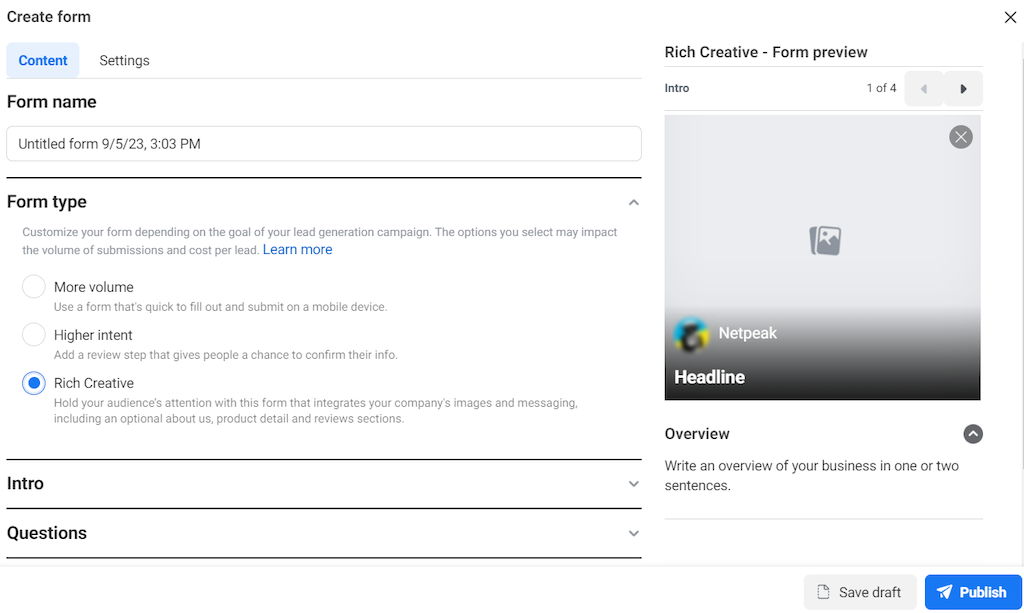This screenshot features the interface of a web application on someone's computer screen. Dominated by a white background with predominantly black text on the left side, the screen displays a structured layout for form creation. 

On the left panel, the title "Create Form" is prominently displayed at the top, followed by a clickable blue box labeled "Content." Adjacent to it is the "Settings" section, which includes a text field named "Form Name" with the placeholder text "Untitled from 9/5/23 3:03 PM." Below this are several horizontal black lines segmenting the form setup options. 

Highlighted in the form type section is an option called "Rich Creative," indicated by a selected blue circle beside it. Further down, sections labeled "Intro" and "Questions" suggest areas where additional information can be input.

On the right side of the screen, there is a gray placeholder box intended for media content, marked with the text "Headline" in the bottom left corner and "Netpeak" in the top left corner.

At the bottom right of the interface, action buttons labeled "Save Draft" in a gray box and "Publish" in a blue box are present, providing options to save or publish the form.